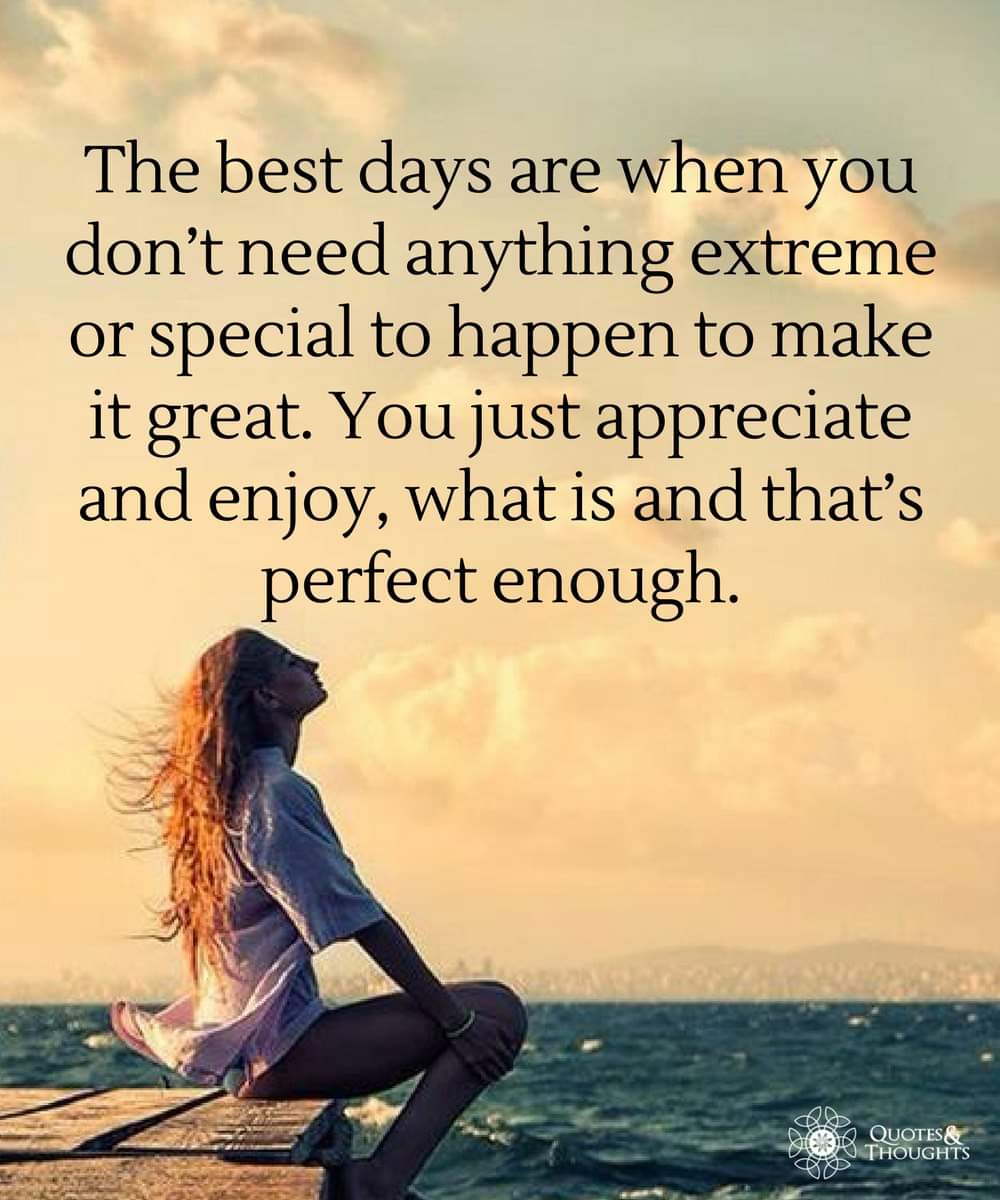In this evocative image, a young woman sits on the edge of a wooden dock, overlooking a vast, choppy body of water with whitecaps. The day is marked by an orange-brown sky filled with billowy clouds, and distant mountains are visible between the clouds and the water. The woman, with red hair flowing over her back, is wearing green tight pants and a purple t-shirt, and she holds her knees, tilting her head upwards with her eyes closed, exuding a sense of peace and freedom. Above her in bold black lettering, an inspirational quote reads: "The best days are when you don't need anything extreme or special to happen to make it great. You just appreciate and enjoy what is and that's perfect enough." The company logo for Quotes and Thoughts is positioned in the lower right corner, adding a final touch to this serene scene.